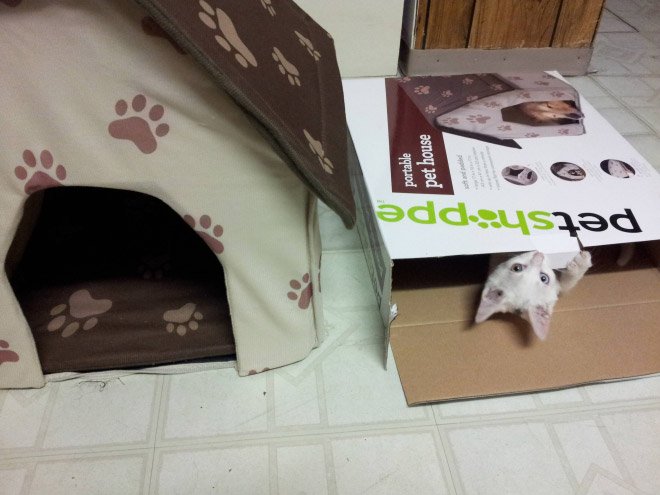The image captures a cozy scene set on a white tile floor within a home. On the left side of the picture, a portable pet house stands assembled, its fabric adorned with light brown paw prints. The pet house itself features an off-white exterior with a dark brown roof and internal floor, spacious enough to comfortably fit a small to medium dog. Adjacent to the pet house lies the open packaging it came in—a white box displaying black and green text, partially readable as "Pet Shop" and "Portable Pet House." Intriguingly, a playful white kitten is seen upside-down, peeking out from the opened box, delightfully emphasizing the cat's curiosity and preference for the box over the intended house. The background includes a partial view of a wall, adding to the casual, homey atmosphere of the snapshot, which appears to be candid rather than professionally taken. The colors in the image span various shades of brown, black, white, gray, light green, and light blue.